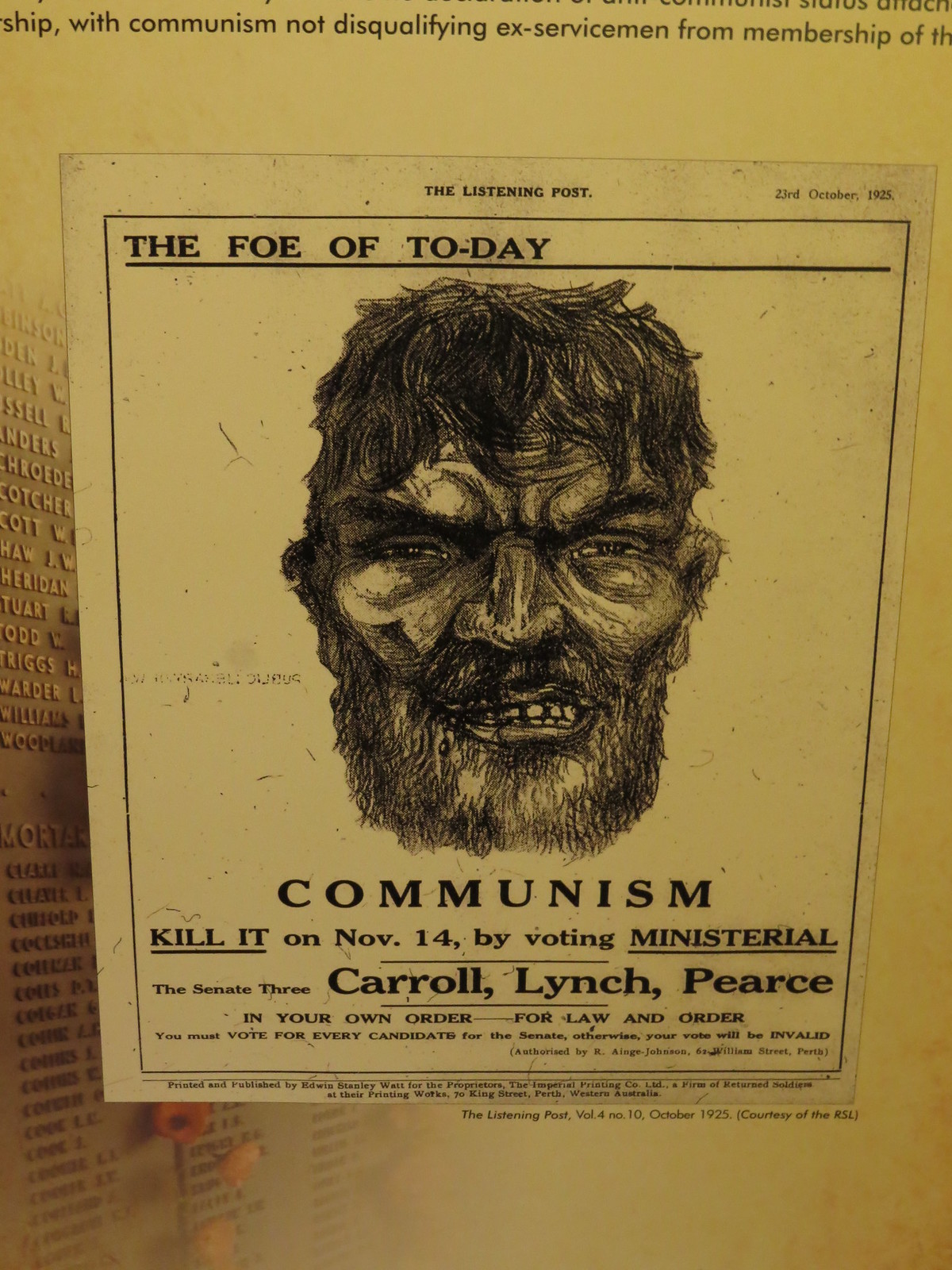The image depicts a vintage political poster with a noticeable yellow background, resembling an aged notification. At the top, the poster is titled "The Listening Post" and dated "23rd October 1925." Below this heading, there's a prominent, wild-looking illustration of a bearded man with hair on his ears, depicting him in an angry, aggressive state, baring his teeth. This caricature is designed to evoke a sense of menace.

The central message of the poster, displayed in bold, gold capital letters, reads: "Communism: Kill it on November 14th by voting Ministerial." The poster urges voters to support law and order by voting for every candidate for the Senate, specifically mentioning three candidates: Carol, Lynch, and Pierce. It warns that failing to vote for every candidate will invalidate the vote.

Additional text at the bottom of the poster states it is authorized by Ainge Johnson of 62 William Street, Perth, and printed and published by Edward Stanley Wait for the Imperial Printing Co Ltd, a firm of returned soldiers at the printing works located at 70 King Street, Perth, Western Australia. The poster is identified as "Listening Post Volume 4, Number 10, October 1925, courtesy of the RSL."

The image appears to be a political advertisement displayed in a museum or memorial, strongly advocating against communism and promoting voting for a specific political party.